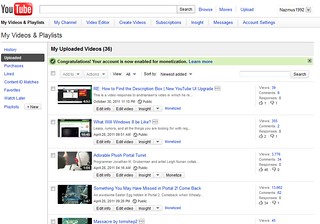The image depicts a YouTube interface with a search bar prominently displayed at the top. The resolution of the image is notably poor, making the details hard to discern. The content on the screen appears to be the user's video management page, showing tabs like "My Videos," "Playlists," "History," "Upload," and more. 

The section labeled "My Uploaded Videos" indicates a total of 24 videos, with thumbnails and information for each video listed. However, due to the blurriness, the text and details within the thumbnails are not readable, even when enlarged. The classic YouTube logo, featuring black, white, and red elements, is positioned in the top left corner.

Additionally, there is a highlighted message in a light yellow-green color starting with "Congratulations," but the rest of the text is illegible. The visible part of the page showcases five video thumbnails, with the fifth one partially obscured at the bottom, suggesting the ability to scroll through more content. The overall color palette of the image includes gray, white, blue, green, yellow, and red.